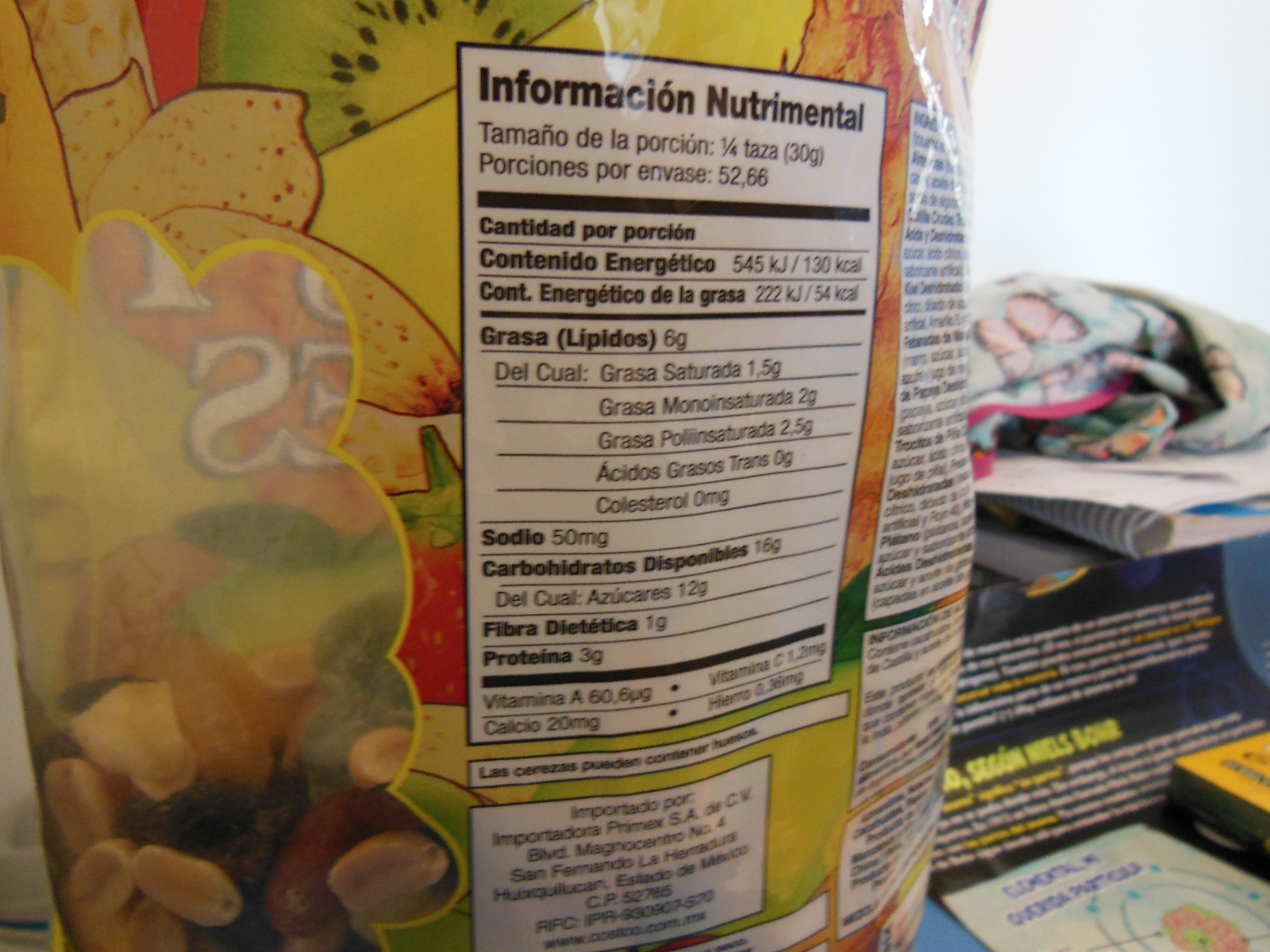This photograph features a detailed close-up of the back of a vibrant, multi-colored food bag, primarily decorated with images of bananas, strawberries, and other fruits. The bag exhibits a yellow, green, red, and dark green palette. In the center of the image, a nutrition label in Spanish is prominently displayed inside a white square with black text. This label provides detailed nutritional information, including calorie content (545 calories, 222 calories), serving size (1/4 taza or 30 grams), lipidos (6 grams), sodium (50 milligrams), and carbohydrates (16 grams per serving). There's a small clear section with a yellow cloud-like outline on the bag, revealing a mixture of nuts, raisins, and other dried fruits such as mangoes and limes. Adjacent to this food bag are various items including a sack of notebooks with white spirals, a cyan blue rag embroidered with hot pink and adorned with pink and orange butterflies, Crayola crayons, and a coloring book.